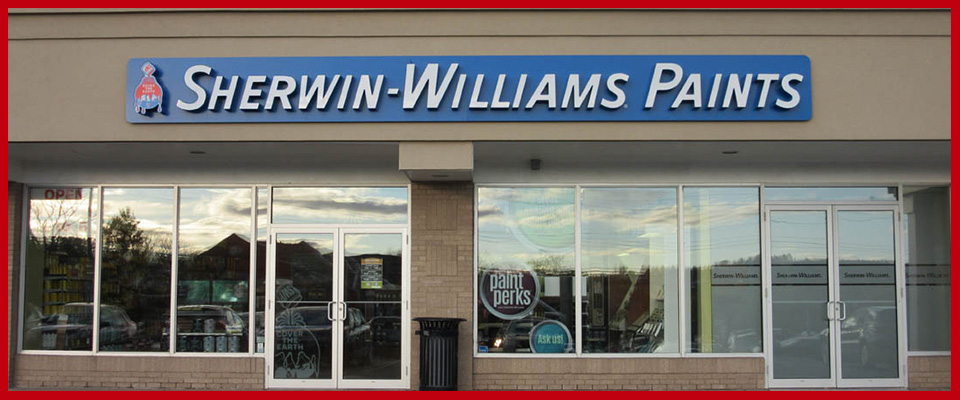The image depicts a vibrant Sherwin-Williams paint store storefront, framed by a striking red border resembling a picture frame that encases the entire facade, enhancing its visibility. The recognizable Sherwin-Williams logo, featuring a paint can with paint spilling over, is prominently displayed in blue with white or slightly grayish lettering. 

The storefront features extensive glass paneling, allowing clear views both into the store and reflections from outside. The entrance comprises two sets of double doors, positioned at both ends of the storefront. Reflections in the windows reveal a bustling parking lot filled with numerous cars. 

A small note adhered to one of the windows reads "Paint Perks," hinting at promotional offers, possibly suggesting that the image was captured during the summer. The sky in the background shows scattered clouds, with one cloud appearing as if it might bring rain.